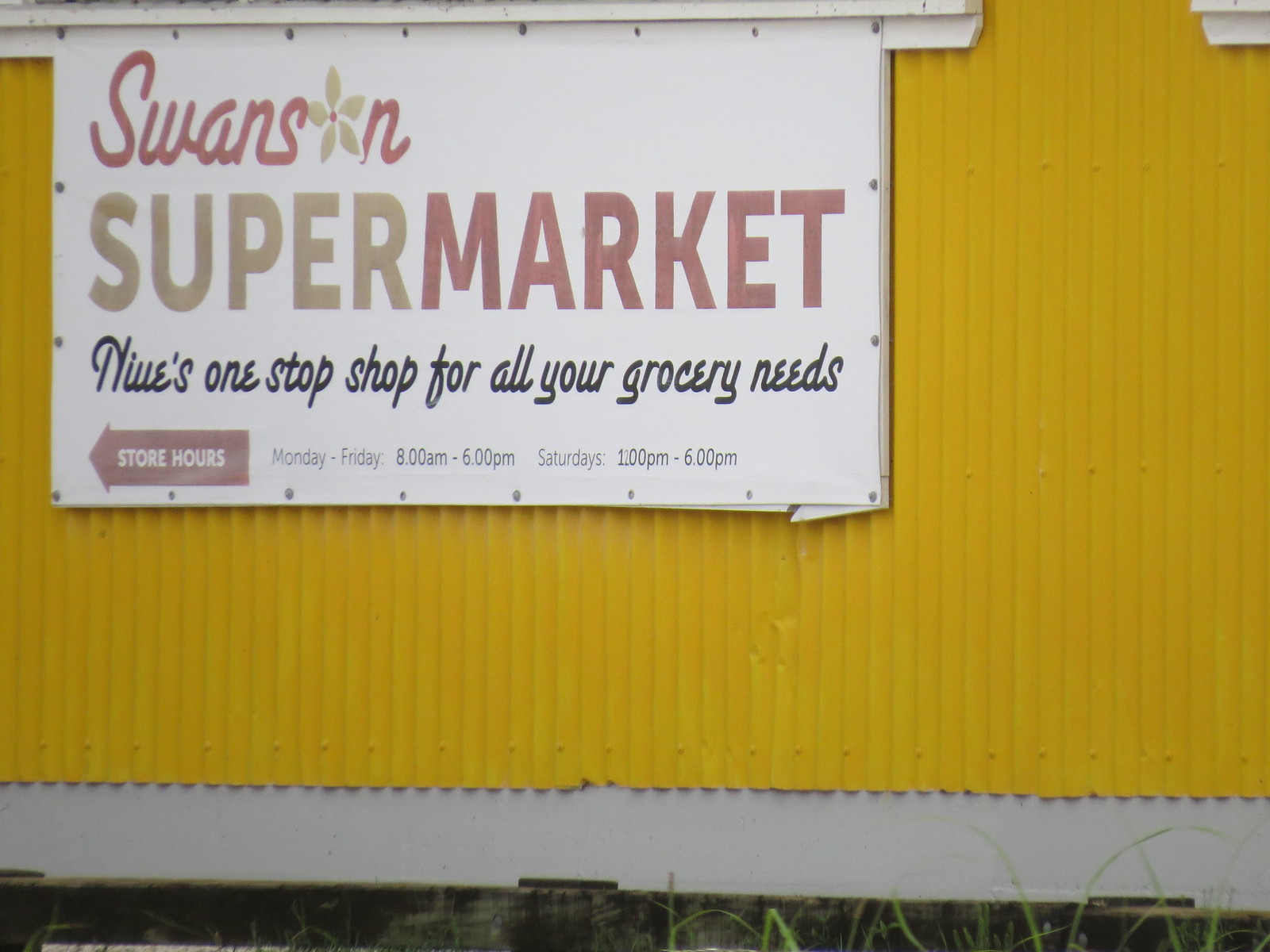In this detailed, color photograph taken in landscape orientation, the primary subject is a side view of a building with a large, horizontally oriented white sign in the upper left corner. The sign, bolted to the building with a bright yellow, corrugated exterior, reads "Swanson" in a weathered, red script with a beige flower replacing the 'O'. Below this, "SUPERMARKET" is written in all caps, with "SUPER" in beige and "MARKET" in red. The text beneath, in black script, states "NEEVES ONE-STOP SHOP FOR ALL YOUR GROCERY NEEDS." 

Additionally, there is a red left-pointing arrow with the store hours listed as Monday to Friday from 8 a.m. to 6 p.m., and Saturday from 12 p.m. to 6 p.m. Visible in the foreground at the bottom of the image is a small patch of grass, enhancing the outdoor daytime setting. The scene includes repetitive elements, such as a white ledge above the sign, which could be part of a window frame, adding to the realistic, photographic representational style of the image. The tones in the image include green from the grass, gray, yellow, tan, black, maroon, and white.